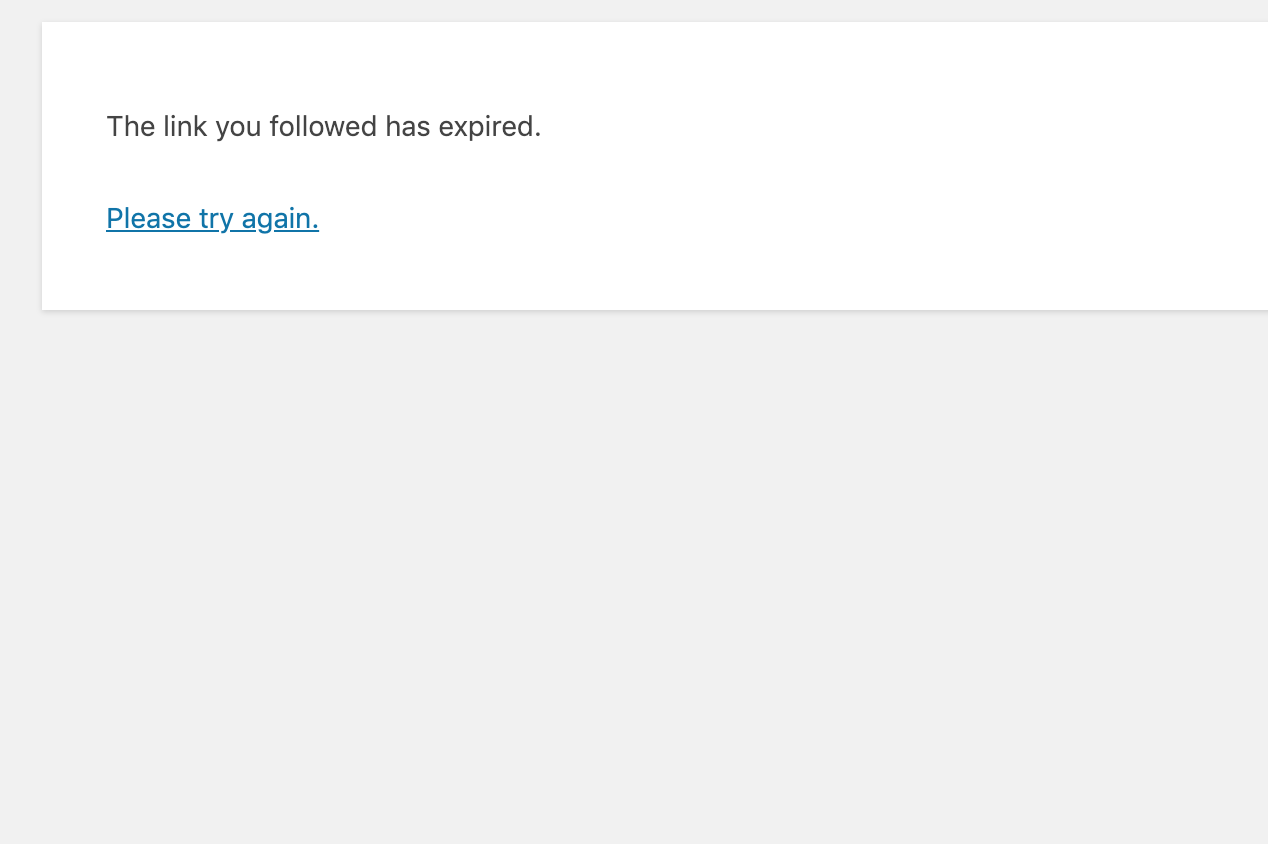This screenshot captures a user interface that could belong to either a computer or a cell phone. The primary focus is a light gray rectangle occupying most of the frame. At the top of this gray rectangle, there is an overlaying white rectangle. Inside this white rectangle, black text reads, "The link you followed has expired." Below this statement, a blue-colored hyperlink text urges the user to "please try again." This indicates that the user attempted to follow a now-defunct link, leading them to this non-functional page. The context of what they were seeking or where they intended to go remains unknown, adding an element of mystery to this otherwise straightforward error message.